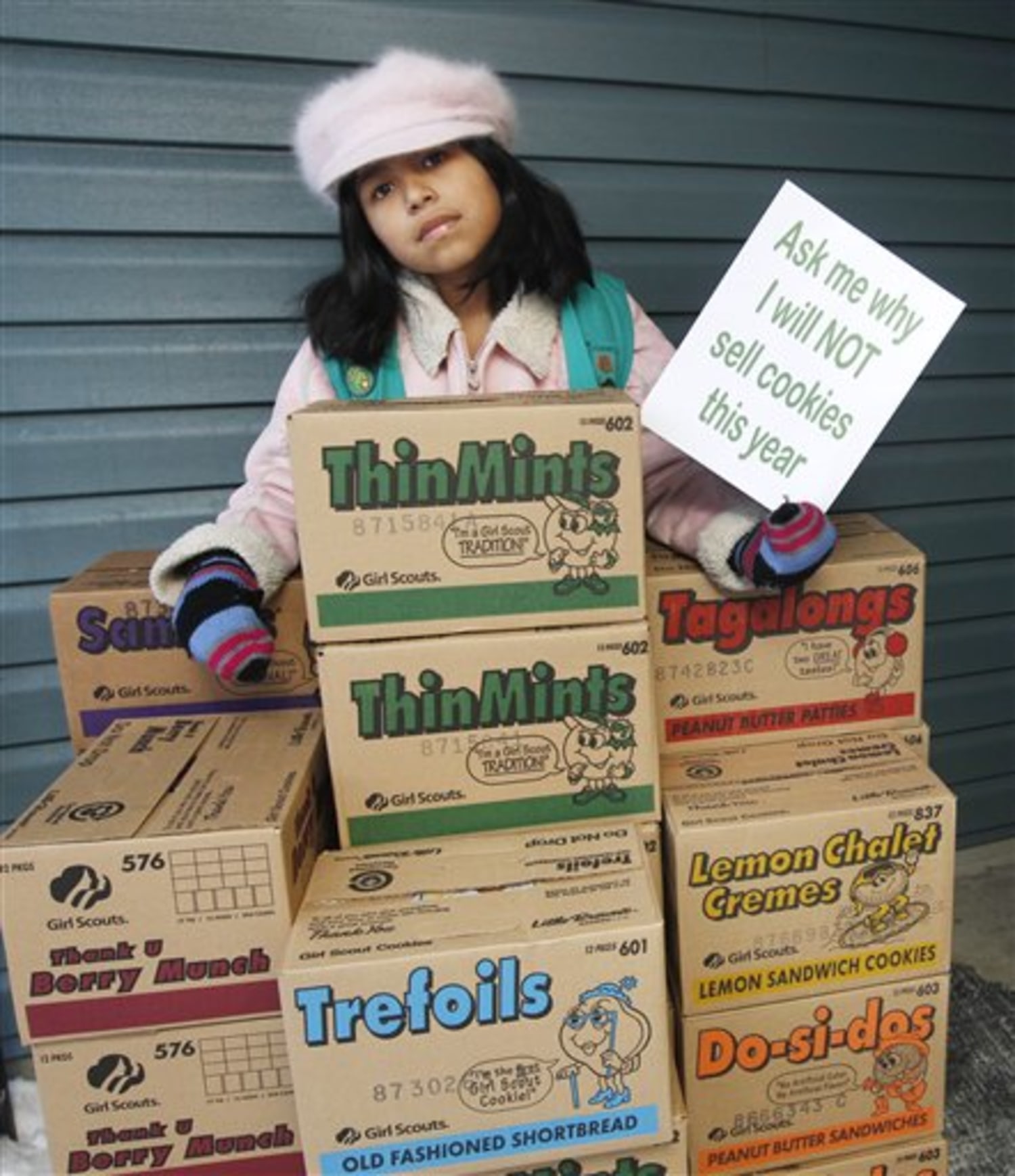The photograph captures a young Girl Scout standing in front of a closed garage door, holding a sign with the message, "Ask me why I will not sell cookies this year." The girl, who appears serious, is dressed in a green vest and a pink fuzzy hat, with mittens on her hands. Her dark black hair falls just below her shoulders. She is surrounded by an array of Girl Scout cookie boxes, stacked from her waist to the bottom of the image. The colorful boxes include recognizable varieties such as Thin Mints, Trefoils (shortbread), Do-Si-Dos (peanut butter sandwiches), Tagalongs (peanut butter patties), Lemon Chalet Cremes, and Thank You Very Much.

The text on the sign is written in green font, which adds to the rustic and somewhat outdated feel of the image, further emphasized by the classic packaging of the cookie boxes. Each box displays a mix of vibrant colors, including shades of red, orange, blue, green, burgundy, purple, gray, turquoise, light pink, black, and white. Some of the boxes also carry additional text and numeric codes, suggesting they are from different production batches.

The composition is a vertical rectangle, with the girl positioned centrally near the top and the cookie boxes neatly arranged in front of her, extending down to the bottom of the photograph. The setting appears to be outside, directly by the garage door, reinforcing the casual, homey atmosphere of the scene.